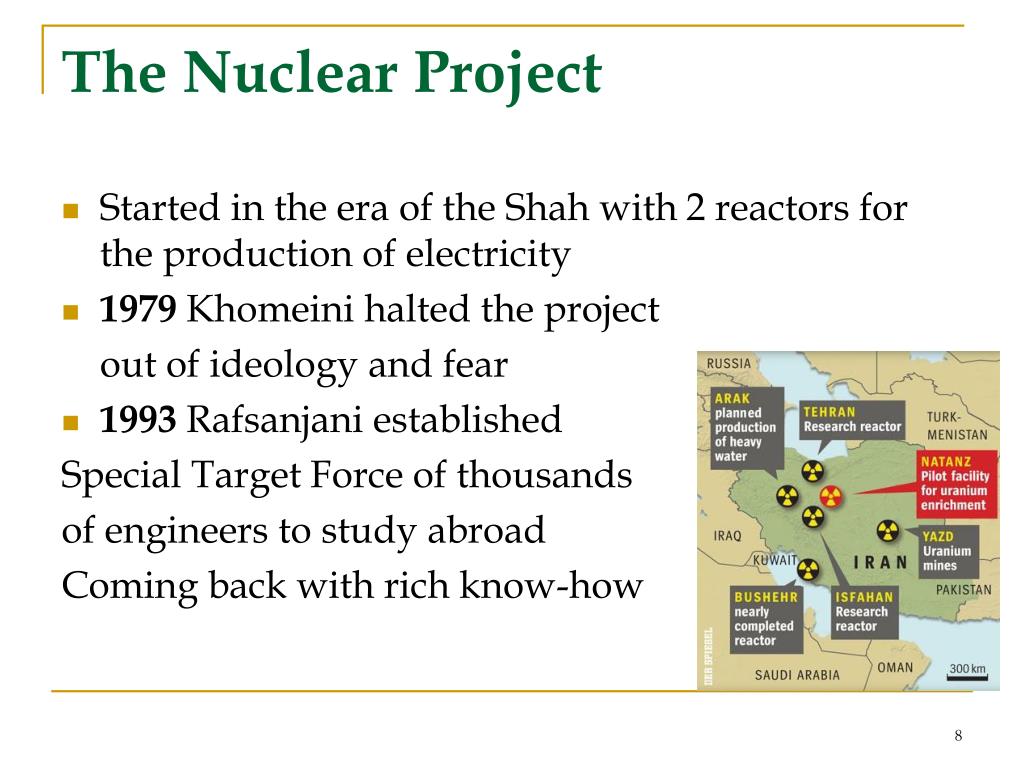The PowerPoint slide, marked as the 8th in the presentation, titled "The Nuclear Project," is bordered in yellow and features green text at the top. It details the historical progression of Iran's nuclear program with three significant bullet points. The first bullet point states that the project began during the Shah's era, establishing two reactors for electricity production. The second point, bolded as "1979," notes that Khomeini halted the project driven by ideological reasons and fear. The third point, noted as "1993" in bold, says Rafsanjani created a special task force that sent thousands of engineers abroad, who returned with extensive expertise. In the lower right corner of the slide is a map of Iran in green, outlined by neighboring countries like Iraq, Saudi Arabia, Oman, Pakistan, Turkmenistan, and Russia. The map highlights several nuclear sites with black and yellow symbols, and a red and yellow symbol. These sites include Arak (plant heavy water production), Bushehr (nearly completed reactor), Isfahan (research reactor), Yazd (uranium mines), and Natanz (pilot facility for uranium enrichment in Tehran).